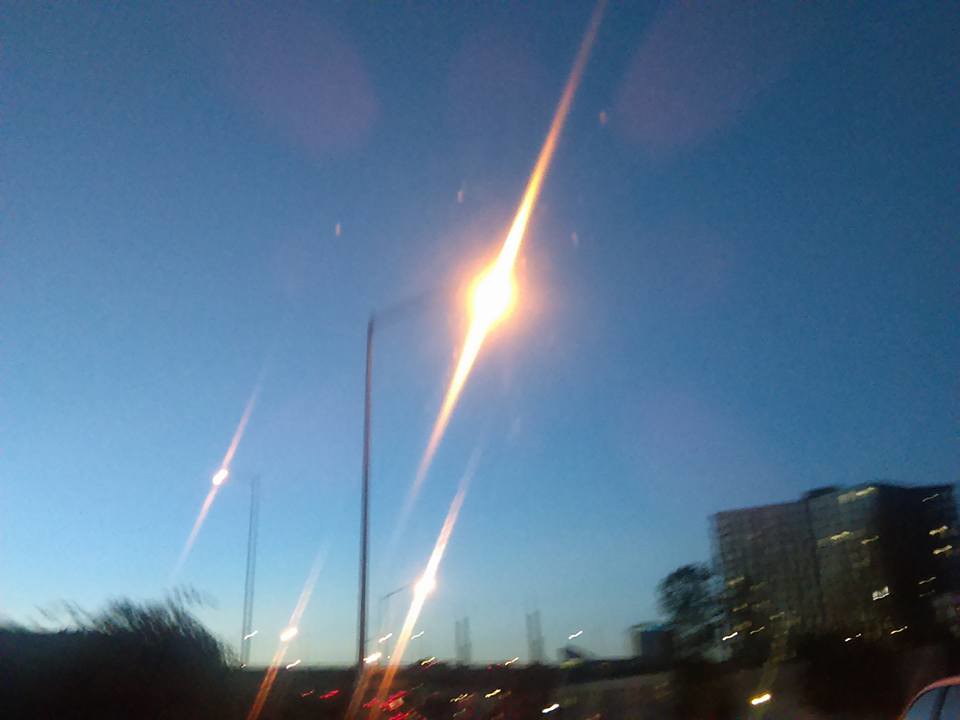The image captures a moment of twilight, either just before sunrise or immediately after sunset, with a sky still cloaked in dim light. The focal point is a series of street lights, creating multiple glares that differ in intensity. These glares are slightly out of focus, adding a dreamy quality to the scene. To the right-hand side of the image, the outlines of several buildings are faintly visible in the background. The majority of the composition is dominated by the expansive sky, which is caught in that fleeting in-between light, neither fully bright nor completely dark. Five distinct glares from the streetlights punctuate the lower portion of the scene, casting subtle reflections and further emphasizing the ambient light of the setting.